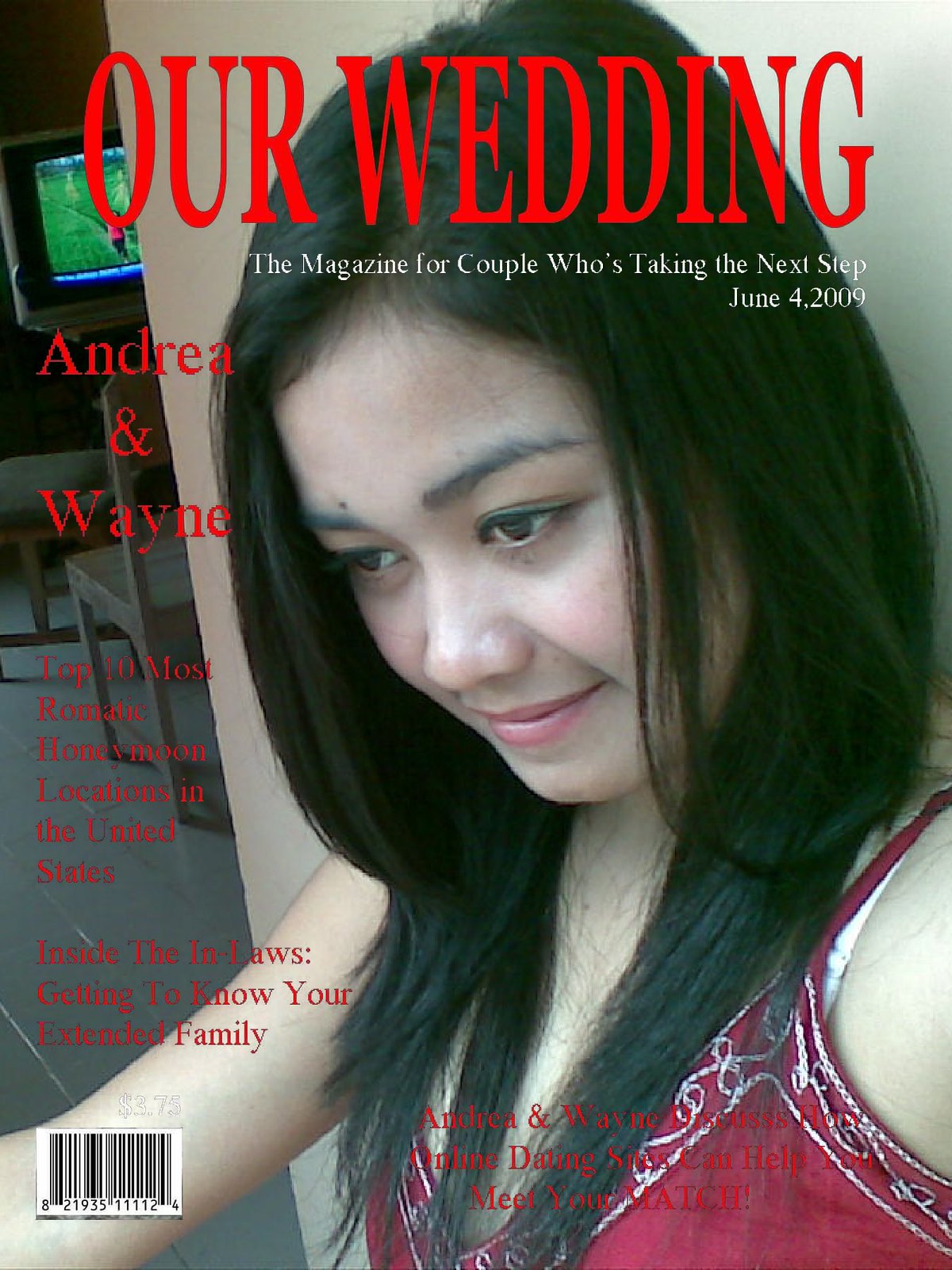The image is the cover of *Our Wedding* magazine, dated June 4th, 2009, designed for couples taking the next step. Dominating the cover is a striking photo of a young Asian woman with dark hair falling just above her breasts. She is wearing a thin-strapped red tank top featuring white designs along the border and appears to be looking down, either concentrating or amused. The background reveals she’s standing against a beige wall, adjacent to a room with grey carpeting and furniture, possibly including chairs and a television with a green screen.

The magazine's title, *Our Wedding*, is prominently displayed in large red letters at the top. Beneath it, the tagline "the magazine for a couple who's taking the next step" and the date "June 4th, 2009" are written in white. To the left side of the cover, more red text reads "Andrea and Wayne." Below that, in smaller red text on a grey background, are features such as "Top 10 Most Dramatic Honeymoon Locations in the United States," "Invite the in-laws: getting to know your extended family," and "Andrea and Wayne discuss how online dating sites can help you meet your match." The barcode is positioned on the bottom left with a price of $3.75 in white text above it.